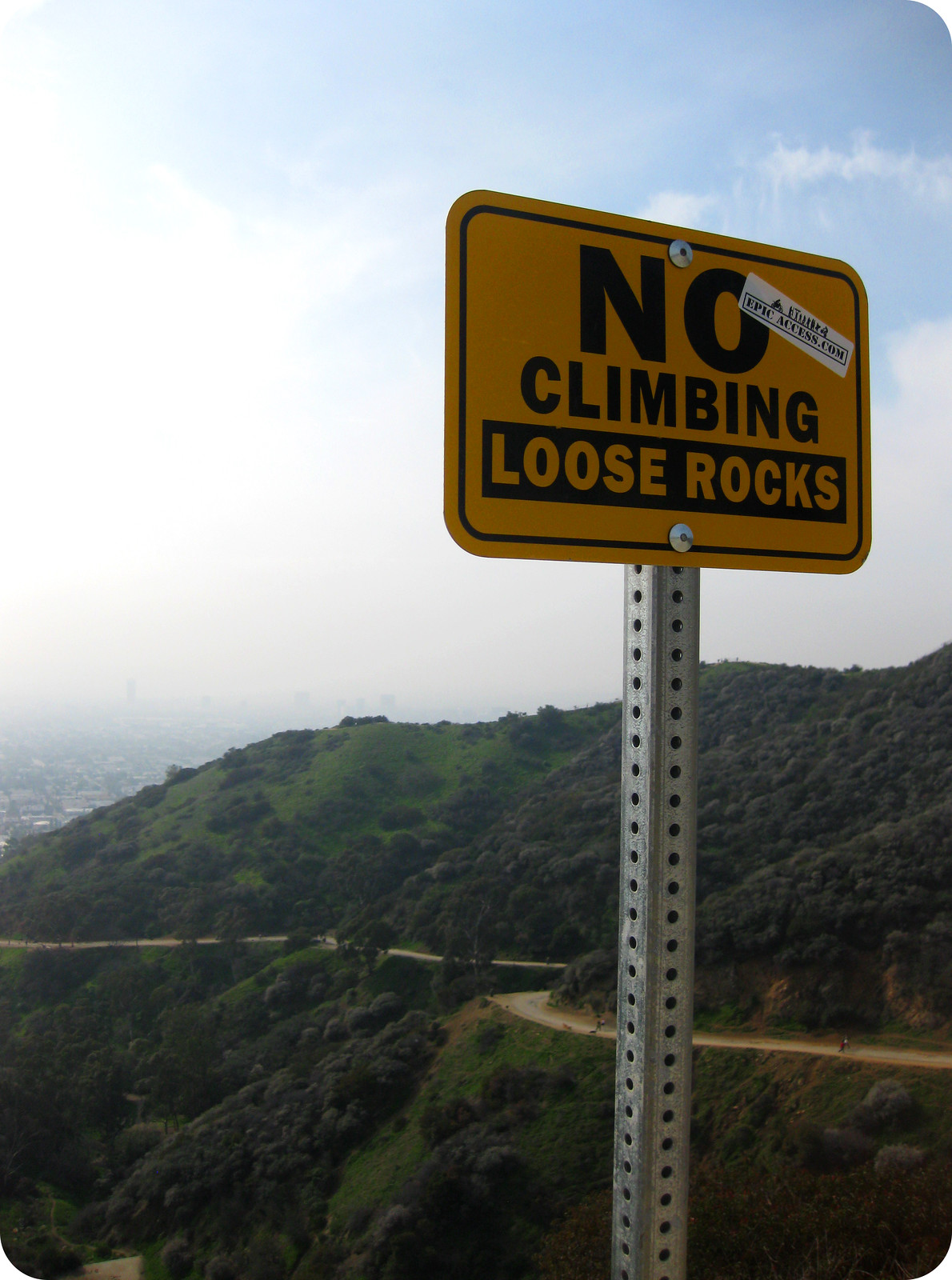This photograph captures a striking scene primarily featuring a roadside sign. The yellow sign with bold black text reading "No Climbing Loose Rocks" is mounted on a robust metal pole, prominently positioned in the foreground. In the backdrop, a deep valley divides the frame, with a ridge covered in dark green vegetation extending beyond. The ridge's narrow highway or trail winds snake-like along its side, populated by small, distinct figures of people suggesting pedestrian use. This trail extends from left to right across the mountainous terrain, hinting at a recreational area, possibly a national park or forest. Distantly, on the left side of the image, diminutive houses peek out, hinting at a nearby settlement. The sky above is a pale blue, partially veiled by clouds through which sunlight streams, casting an idyllic daytime glow over the scene.